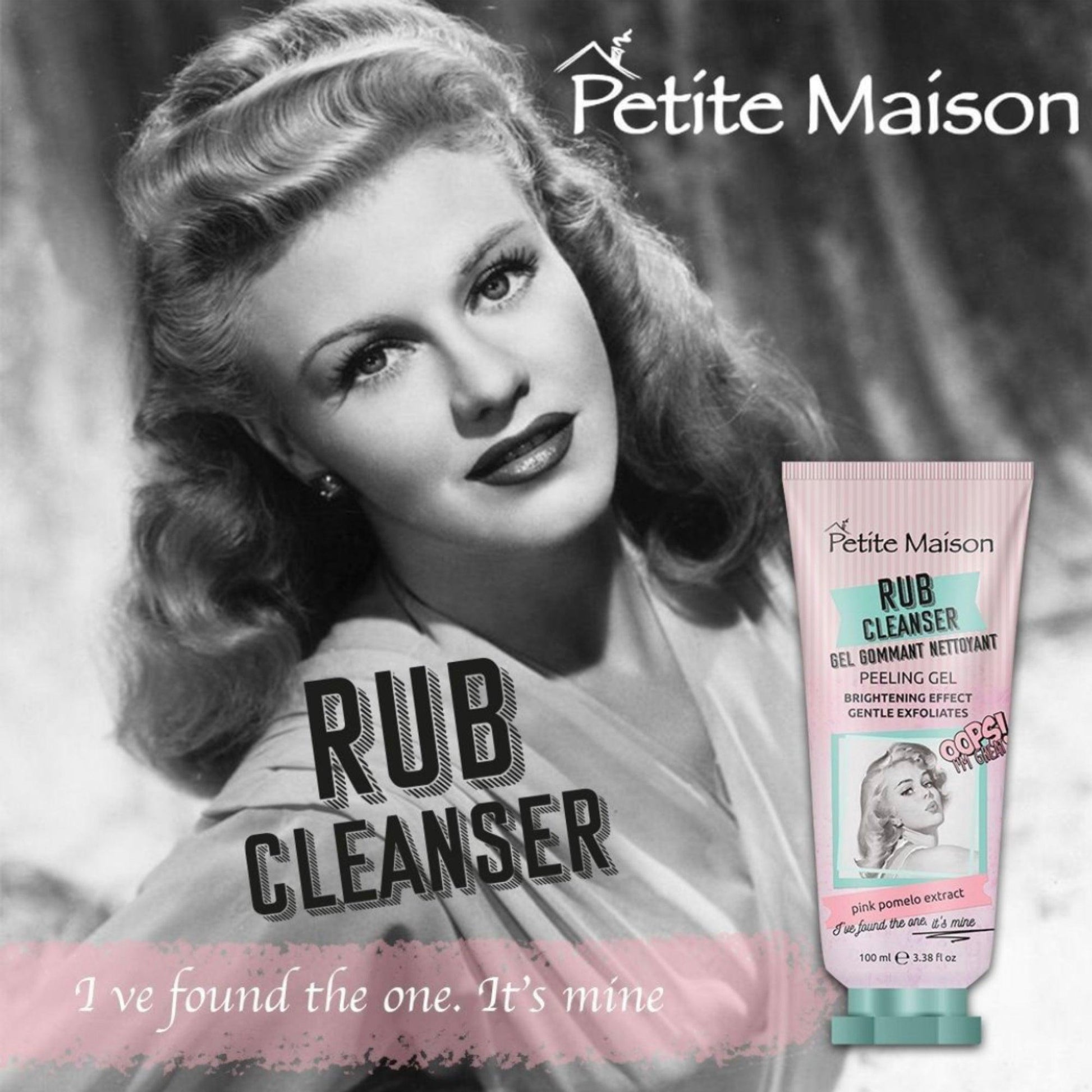This advertisement for a skin cleanser prominently features a black and white photograph of a celebrity from the early 1900s, who is posing elegantly and gazing directly into the camera, her wavy hair cascading past her shoulders. In the top right corner, the ad displays "Petite Maison" in white text, complete with a chimney design above the 'P'. At the bottom left corner, bold black text reads "Rub Cleanser". Overlaying the photograph, a semi-transparent pink banner with white text states, "I found the one. It's mine." In the bottom right corner of the ad, there is an image of the beauty product itself, a pink and white striped tube labeled "Petite Maison Rub Cleanser Gel Gommant Nettoyant Peeling Gel", and indicating its brightening effects and gentle exfoliating properties with Pink Pomelo Extract. The tube also features a green-capped top and a black and white photograph of a different celebrity framed with a green border.